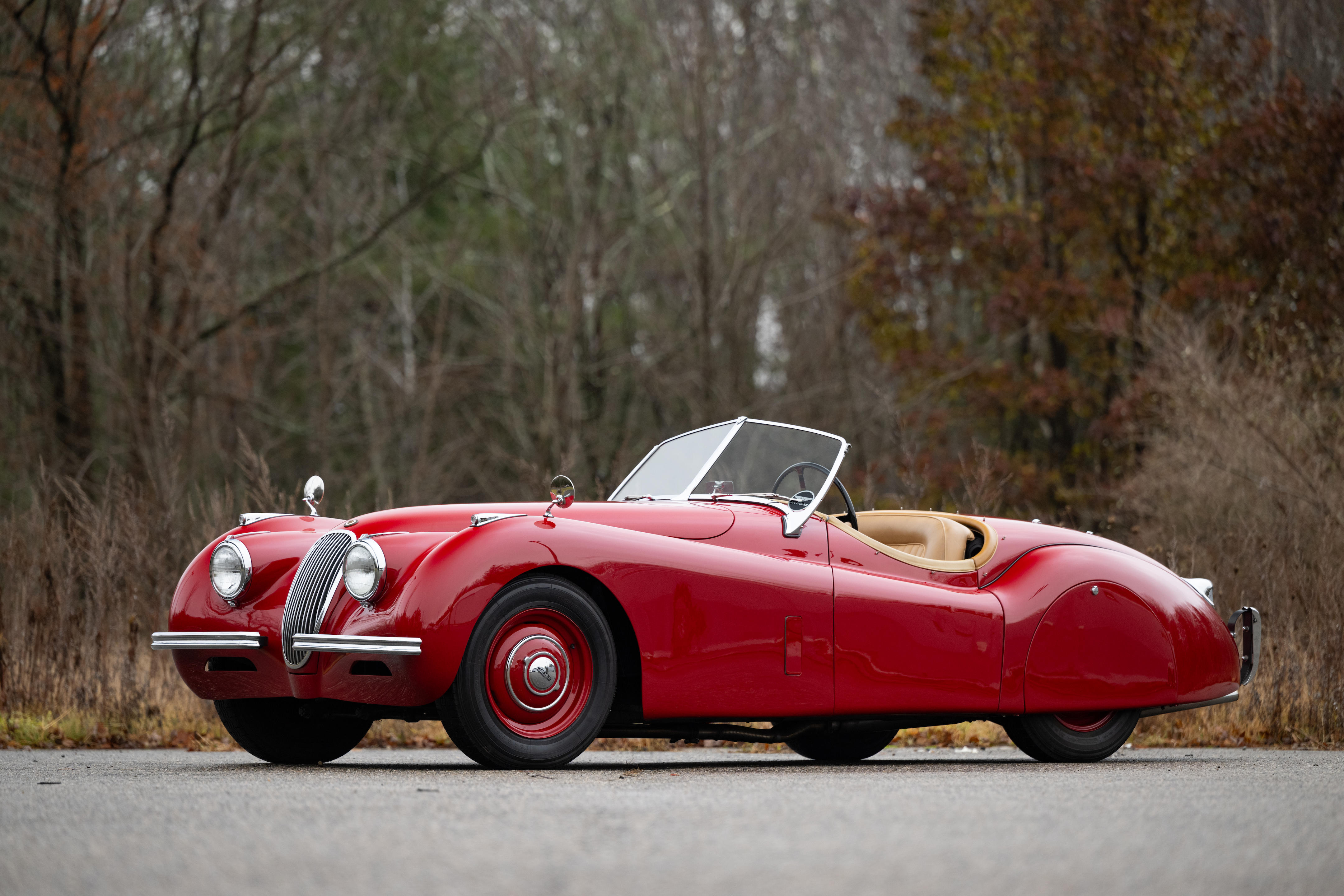This photograph captures a striking vintage red car, evocative of luxury models from the 1930s or 40s. The car is distinguished by its streamlined, curvy, and low-profile design, featuring a single row of cream leather seats. The vivid red extends to its rims which complement the black tires. Notably, the rear wheels are partially shrouded by the car's body, adding to its stylish appearance. The car's open-air coupe design suggests that if it has a convertible roof, it is neatly tucked away. A thin steering wheel is positioned on the left side, suggesting Western standards.

The setting is a cloudy late fall or winter day on a plain asphalt road, flanked by a dense forest of bare or partly green trees, indicating the season. The absence of a driver and the car's central focus in the frame hint that the photograph emphasizes the vehicle itself, celebrating its unique and opulent features. The backdrop of autumn leaves and bare trees, combined with a small, rounded front grille with silver accents and a slightly curved backward windshield, further enriches the vintage allure of this remarkable automobile.